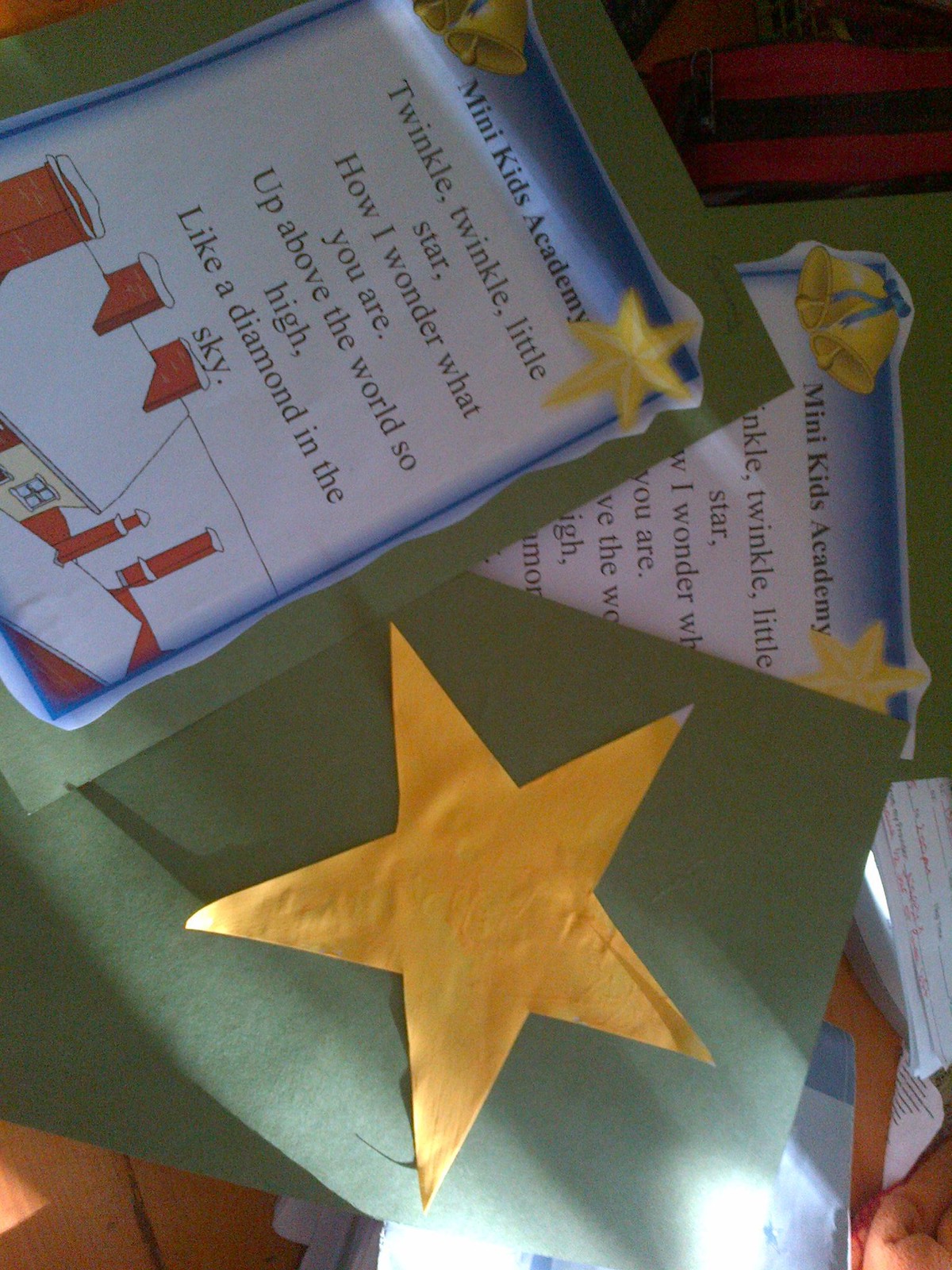The image displays a charming, homemade card likely crafted by a child using green construction paper. The primary card, situated on the left, features a printout glued on top. This printout has a gradient blue border and contains the text, "Mini Kids Academy" and the nursery rhyme, "Twinkle, twinkle, little star, how I wonder what you are. Up above the world so high, like a diamond in the sky." Above the text are yellow bells on the top left and a yellow star on the top right. Below the text, there is an illustration of snow-covered rooftops with three chimneys. Positioned beside this main card is another piece of green construction paper featuring a large yellow star cutout. The cards are organized in a slanted manner from left to right as if placed casually on a tabletop, with an identical card to the first one lying beneath both. The overall presentation evokes a whimsical, storybook-like quality.